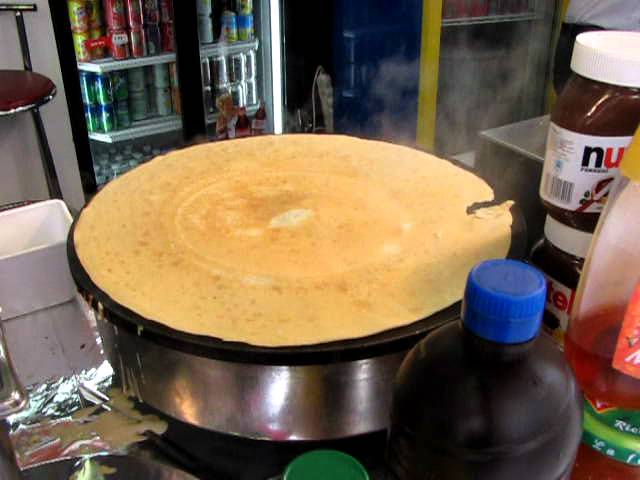This photograph captures a bustling restaurant kitchen scene centered around the preparation of a crepe. At the forefront, a golden crepe, slightly torn on one edge, cooks atop a silver, chrome-colored cylindrical crepe maker with a black circular cooktop. Surrounding the crepe are various jars and bottles, most notably two stacked jars of Nutella tilted to reveal parts of their labels ("NU" on the top jar, "TE" on the bottom jar). A dark bottle with a blue cap is also visible in front of the crepe maker, alongside other sauces and condiments. In the background, a cooler stocked with an array of soda cans, including Sprite and Dr. Pepper, anchors the kitchen setting. Aluminum foil and a container with a green lid add to the sense of a busy culinary workspace.